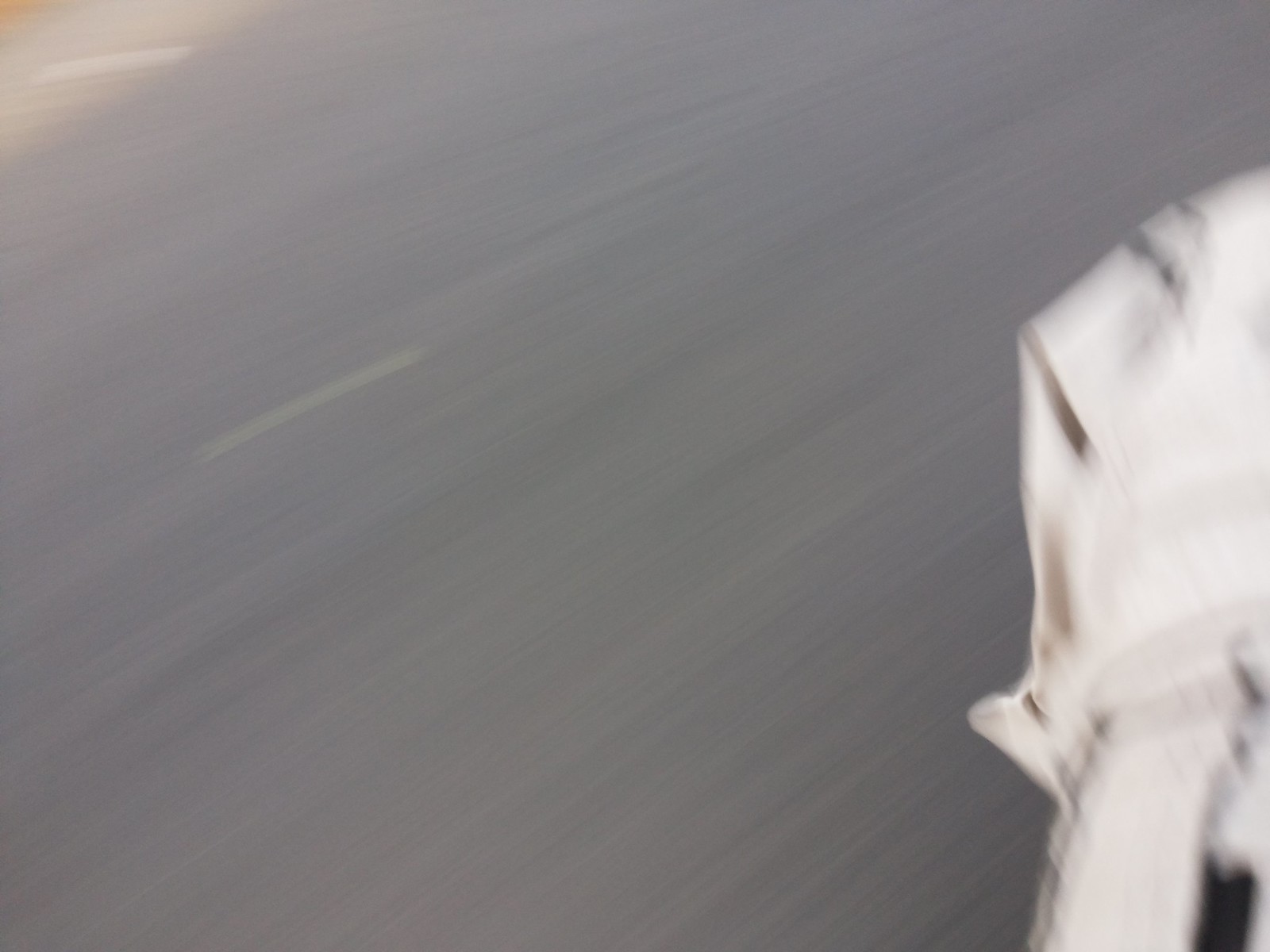This photograph captures a striking scene enveloped in a dramatic motion blur, evoking a sense of swift movement or long exposure. Dominated by a light grey palette, the image is energized by a warm, yellow-orange glow emanating from the top left corner, casting a subtle gradient across the frame. Along the right side, a blurred white object with indistinguishable black markings hints at a large form, possibly a piece of clothing, though its definitive nature is obscured by the motion. The extensive blur across the image creates a visual effect reminiscent of night sky photography, where stars streak into trails as if captured at high speed, imbuing the scene with an ethereal, almost otherworldly atmosphere.